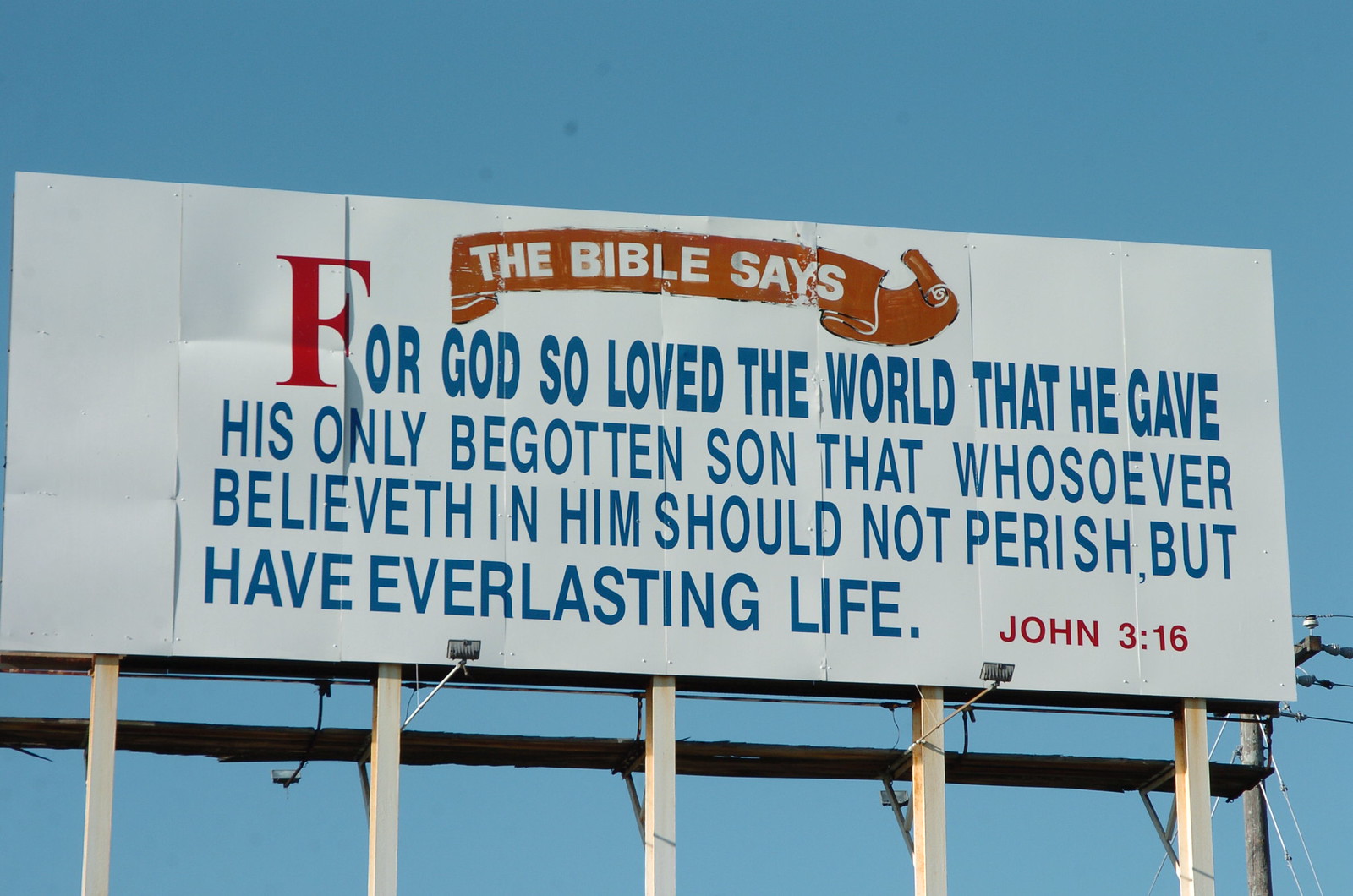A large outdoor billboard stands proudly against a vivid, clear blue sky, with not a cloud in sight. The billboard is predominantly white, adorned with blue text, and features a striking red banner across the top. The banner reads in white text, "The Bible says:" Underneath, in blue, is a prominent scripture: "For God so loved the world that He gave His only begotten Son, that whosoever believeth in Him should not perish but have everlasting life." In the lower right corner of the billboard, the citation "John 3:16" is boldly written in red text. This impactful message is supported on five sturdy white pillars. While the back of the billboard hints at additional content, it's obscured from this view. In the lower right corner of the image, the base of a power pole with faintly visible power lines subtly intrudes, framing the scene.